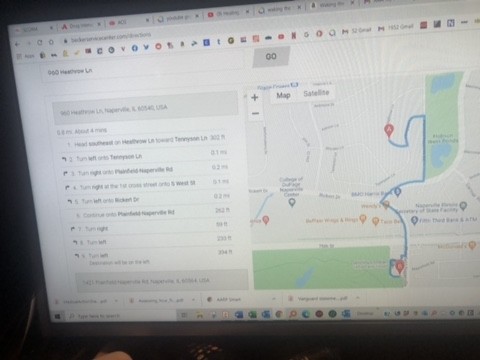This color photograph depicts a highly blurry image of a computer screen. On the right side of the screen, a map can be seen, featuring a mixture of gray, green, and blue hues, while on the left, a set of directions is displayed on a white background with black text. The route on the map is highlighted in dark blue and marked with a red pin at each end. The overall image is extremely blurry, making specific details nearly indiscernible. Surrounding the photograph is a black border. Scattered across the computer screen are various colors, including yellow, blue, green, orange, and gray, though their exact purpose is unclear. Notably, on the bottom edge of the image, towards the left (but not in the corner), there's a peach-colored area that resembles a skin tone.